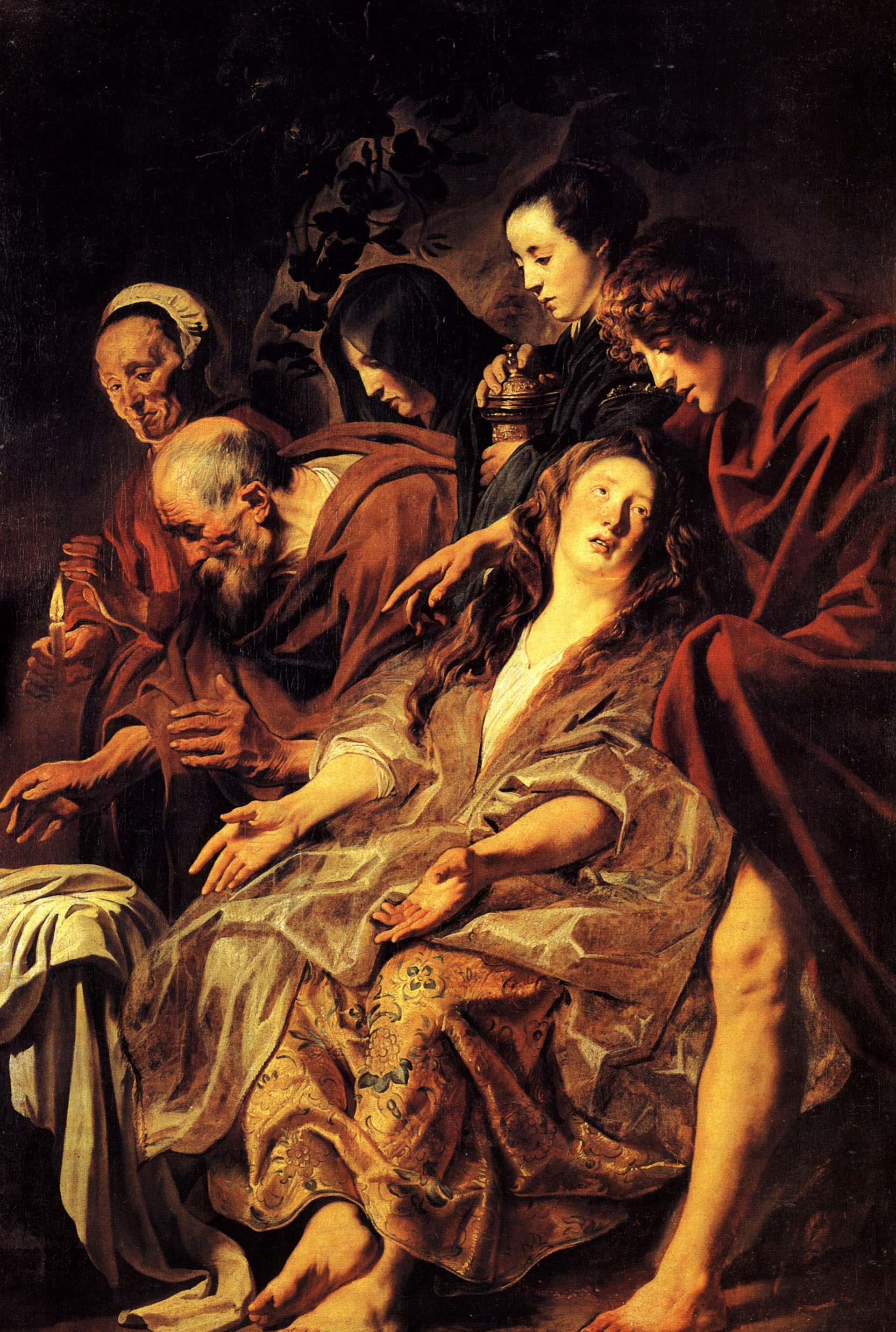The painting, possibly dating back to the 16th or 17th century and evocative of the Dutch masters like Vermeer or Van Eyck, depicts six figures in a dark, moody background typical of the period. Central to the image is a young woman who appears ill or in distress, draped in cream-colored clothing and a shawl, her expression agonized and hands open. She is barefoot and seated, surrounded by five individuals, at least three of whom are clad in brown robes suggesting they could be monks or religious figures. One woman among them has a white bonnet, and another has dark hair. The figures' attention is directed towards an area to the left of the frame, off the depicted scene, possibly at a table covered with a cloth, from where the group seems to draw a collective focus. Amidst the somber atmosphere, the figures' concern and the intricate details of their attire hint at a larger, unseen narrative.